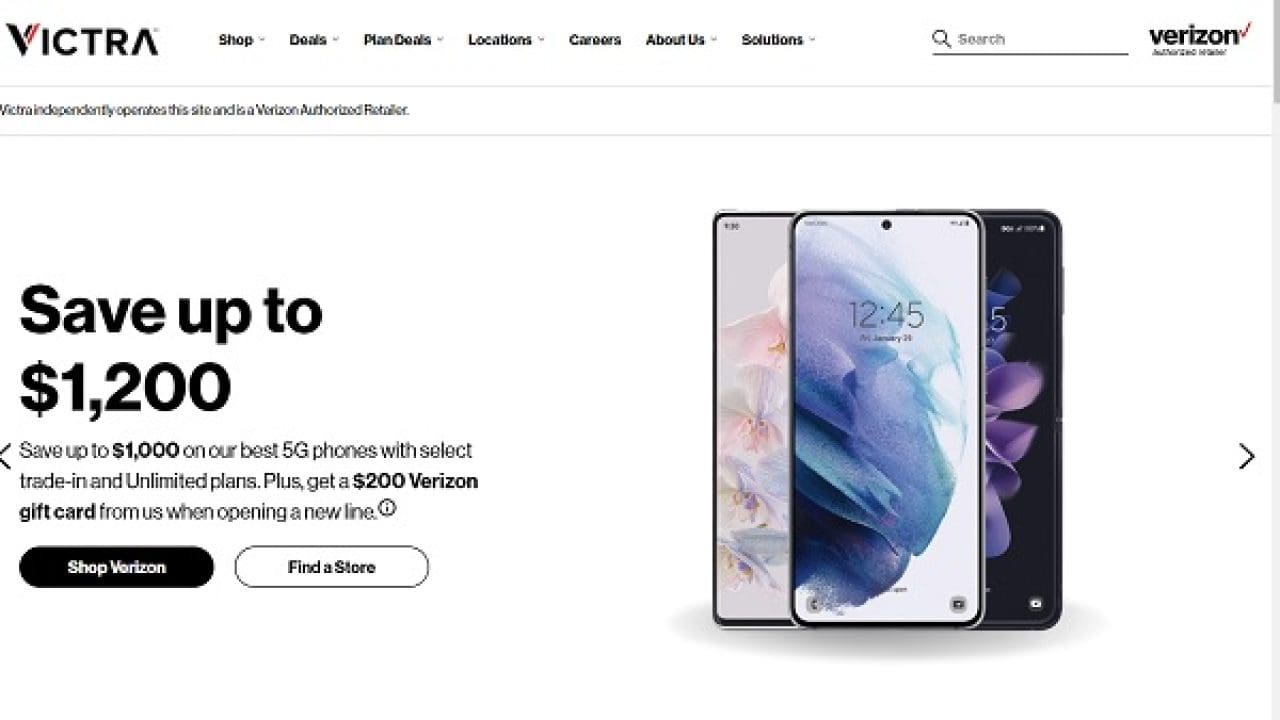This screenshot, taken from the Victra partner section of the Verizon website, highlights a promotional offer. At the top of the page, the header features navigation links to key sections: Shop, Deals, Plan Details, Locations, Careers, About Us, and Solutions, with the Victra logo prominently displayed in the top left corner. The top right corner houses a search bar followed by the Verizon logo.

The main section of the page showcases three smartphones arranged with the central phone fully visible, flanked by partially obscured phones on each side. Each device displays a vibrant, colorful background on its screen. To the left of the phones, a promotional text announces substantial savings: "Save up to $1,200, save up to $1,000 on our best 5G phones with select trade-in and unlimited plans, plus get a $200 Verizon gift card from us when opening a new line." Below the text, two call-to-action buttons are displayed: a black "Shop Verizon" button and a white "Find Store" button.

On the far right side of the page, a navigation arrow button hints at more images, and a scrollbar runs vertically along the edge, inviting users to explore further.